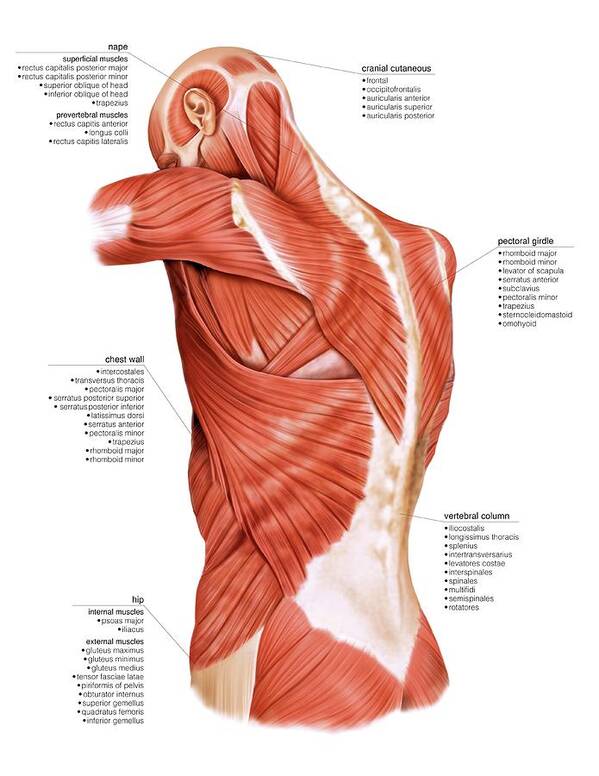This detailed illustration depicts the muscular anatomy of a human male from a posterior view, starting at the top of the head and extending down to the upper glutes. The entire backside appears to be stripped of skin to expose red muscle fibers interspersed with white spots, giving a vivid representation of the musculature. The top of the head is rounded, and a light beige-colored ear is visible. Labels are meticulously applied to various muscle groups including the nape (back neck area), cranial, pectoral girdle, chest wall, vertebral column, and hip. The image suggests a highly athletic physique, with the musculature showcased as enveloped in a sheen of white fat, enhancing the depth and texture of the illustration.